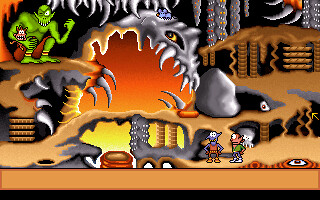In this nostalgic, pixelated image, seemingly derived from a classic computer game, we observe a detailed and vibrant scene. The illustration is oriented in portrait mode and boasts a palette dominated by shades of orange, gray, brown, and yellow. 

In the upper left corner, a prominent green creature with a furious expression grabs attention. Despite having a muscular build, this character sports noticeably thin arms and is tightly clutching a smaller, red-colored creature, which appears to be in distress, possibly screaming.

Amidst the chaos, fragments resembling parts of a gray dragon are scattered throughout the composition, including discernible gray claws and a sizable gray boulder. 

At the bottom of the image stand two figures, each with their hands placed firmly on their hips, their postures exuding concern or contemplation as they survey the scene unfolding before them. Together, these elements weave a rich tapestry of drama and tension, evocative of the early days of computer gaming.